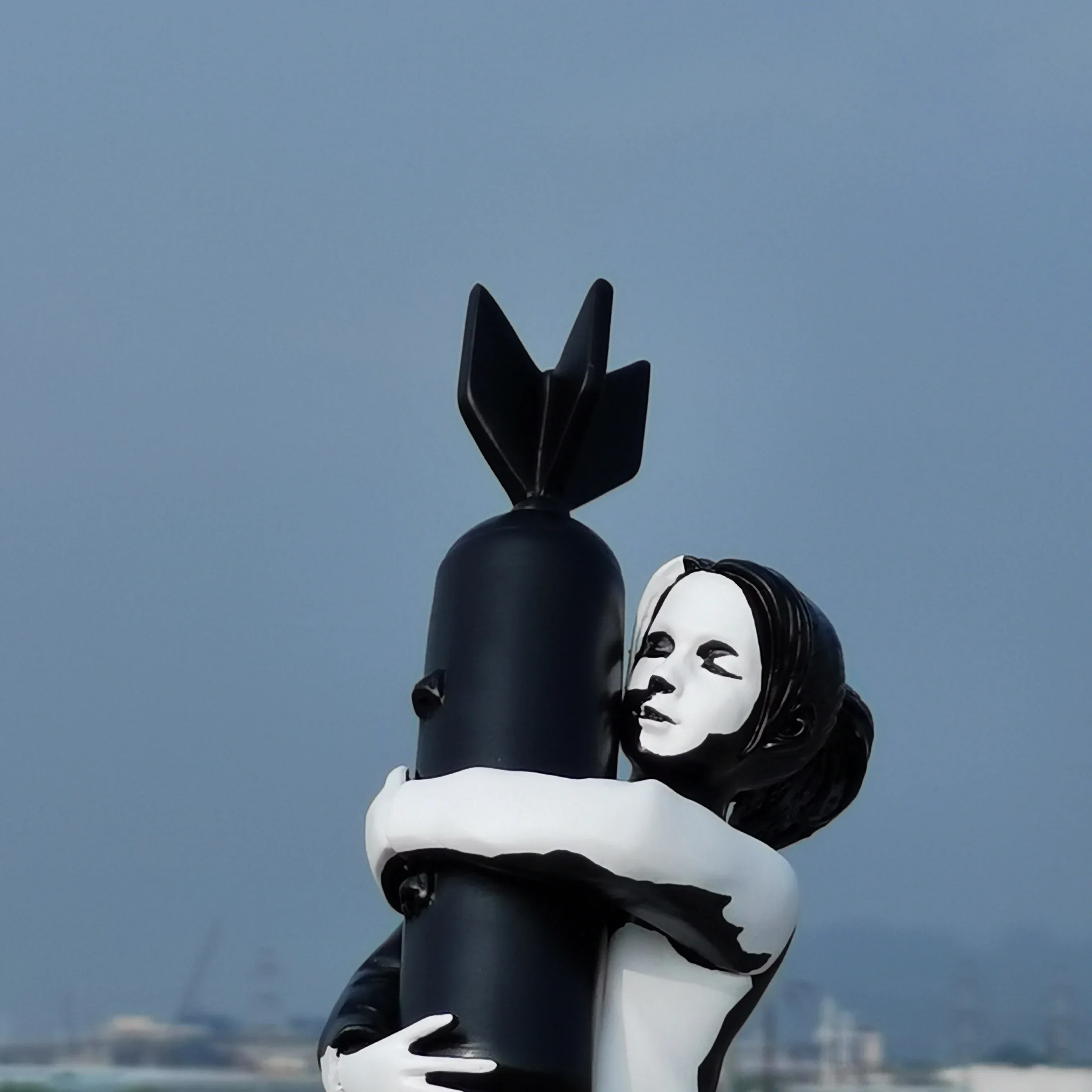This striking photograph features a modern sculpture by Banksy, showcasing a reflective chrome statue of a young girl with black low lights accentuating her hair and shadows. The figure is portrayed in an embrace with a black vertical torpedo, fins at the top, evocative of a bomb. Her face, with eyes mostly closed and mouth partially open, is pressed close to the torpedo, creating an ironic and poignant scene. The sculpture is positioned centrally and extends to the middle bottom of the image. The background presents a light blue-gray sky and an out-of-focus industrial landscape, reminiscent of a marina area, blending the realistic details of a photograph with the intricate artistry of the sculpture. The composition captures a stark contrast between the innocence of the young girl and the menacing presence of the bomb, all rendered in a mixture of whites, blacks, grays, and light blues.